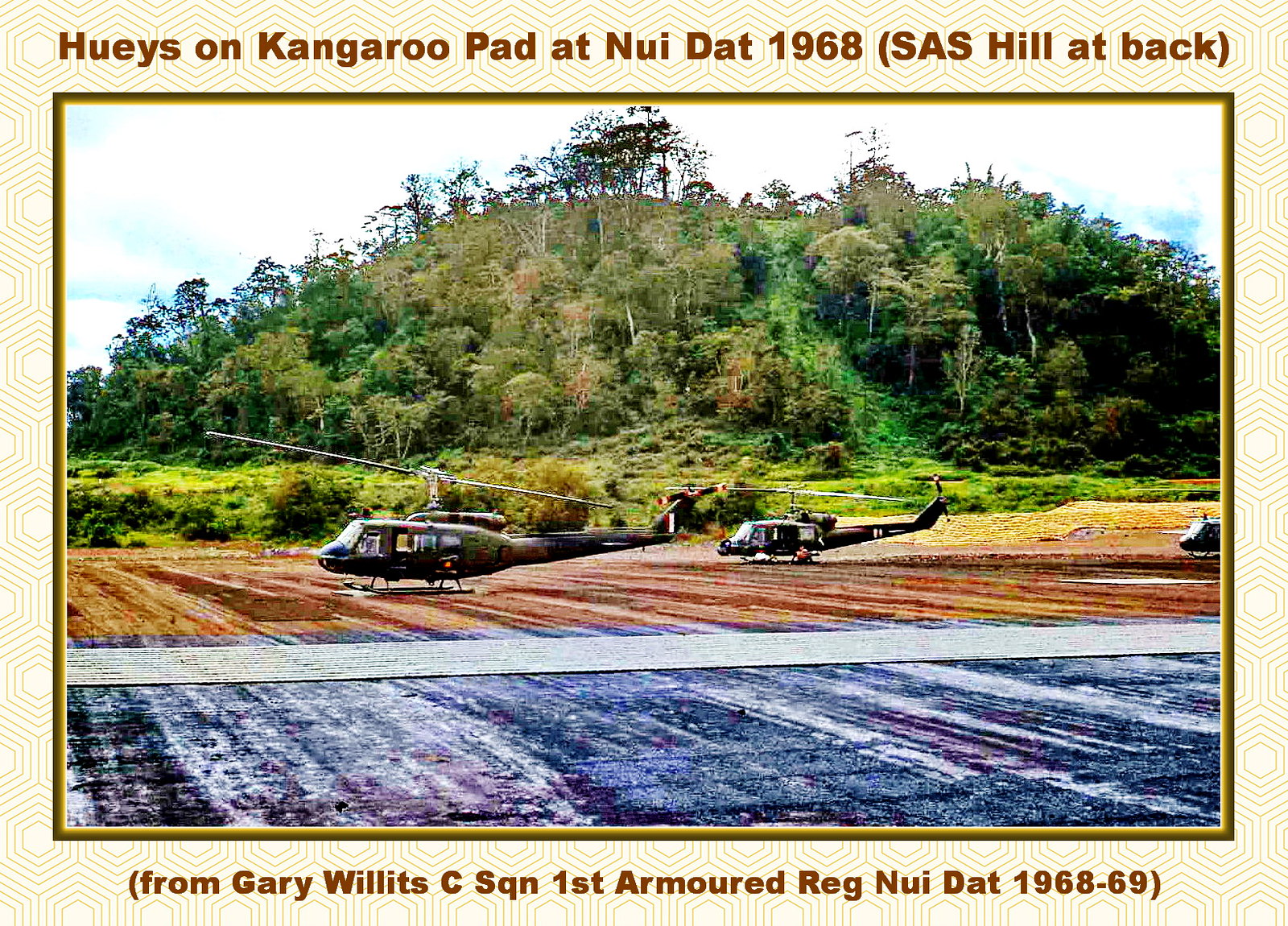This color photograph, taken during the Vietnam War in 1968, features two UH-1 "Huey" helicopters stationed on Kangaroo Pad at Nui Dat. Both helicopters are viewed from the side, with their noses pointing to the left and tails to the right, positioned on a dirt field. The helicopter on the left is closer to the viewer than the one on the right. The image background showcases a field with an airstrip, a dense cluster of trees, and a mountainous terrain beneath a mostly cloudy sky. The top caption reads: "Hueys on Kangaroo Pad in Nui Dat, 1968 (SAS Hill at back)." The bottom caption, in smaller text, reads: "From Gary Willits, C-Squadron, First Armored Regiment, Nui Dat, 1968-69." The photograph illustrates the iconic UH-1 helicopters, colloquially known as "Hueys" due to their original Army designation HU-1, reflecting their pivotal role in utility operations during the conflict.